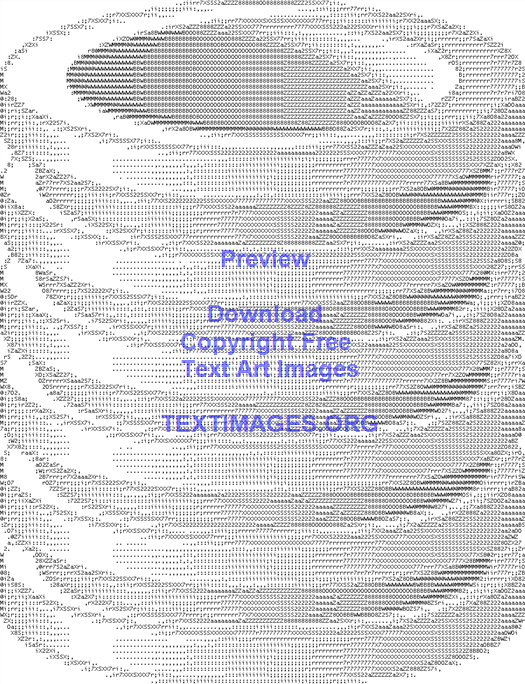The image is a detailed, computer-generated ASCII art depicting a stack of concentric rings, alternating between larger and smaller sizes, mimicking the appearance of a screw thread. The rings, composed of repeating symbols, create a layered effect of alternating light and dark shades of gray. In total, there are six larger rings and five smaller ones, arranged in a pattern of larger, smaller, larger, smaller, and so on. Superimposed over this intricate backdrop is semi-transparent blue text, centrally located, that reads, "Preview, download, copyright-free text art images, textimages.org," written in a sans serif font. The entire composition rests on a stark white background, creating a striking visual contrast.